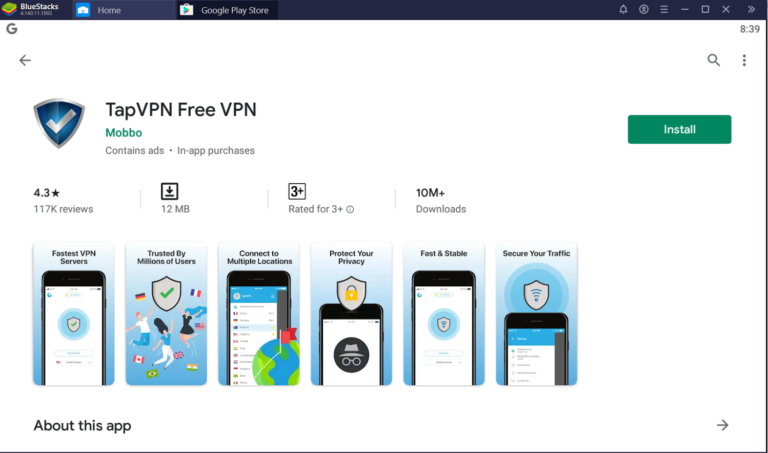A detailed and cleaned-up caption for the image could be:

---

Screenshot of a desktop browser displaying the Google Play Store page for the app "TapVPN, FreeVPN." The background of the page is white. On the left side, there is a large shield icon featuring a checkmark. To the right of this icon, the app's name "TapVPN, FreeVPN" is displayed in large black letters. Below that, the developer's name "Mobo" is visible in green lettering. Further down, it indicates in small grey letters that the app "Contains ads" and offers "In-app purchases."

On the far right side of the page, there is a prominent green rectangular button labeled "Install." To the left of this button, the app's rating is shown, which is 4.3 stars based on 117,000 reviews. Next to the rating, there is a download icon followed by the size of the app, which is 12 megabytes. To the right of this download information, there is a square icon indicating the app is "Rated for 3+."

On the extreme right of the page, the number of downloads is displayed, showing "10 million downloads." Towards the bottom left of the page, there are several landscape-oriented screenshots of different screens within the app.